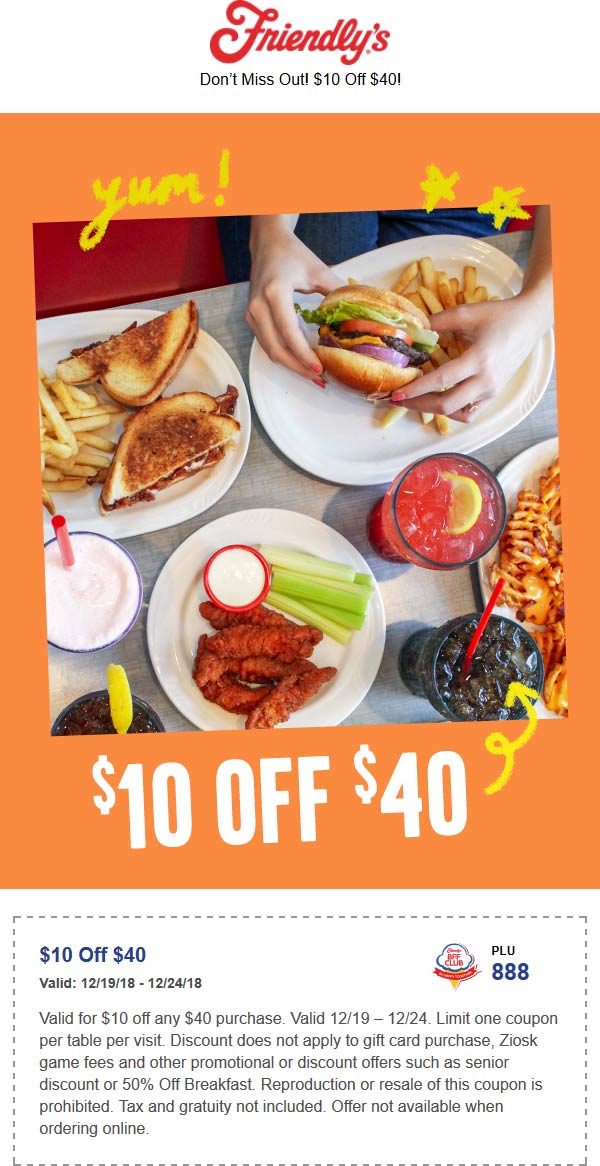Here is a detailed and cleaned-up caption for the image described:

"This is a vibrant advertisement from Friendly's featuring their latest promotion. At the top, the iconic Friendly's logo, presented in a distinctive red stylized script font, immediately catches the eye. Beneath the logo, bold text reads 'Don't Miss Out' accompanied by the promotional price of $10.40. The centerpiece of the ad is a mouth-watering image of a table laden with an assortment of appetizing dishes. One plate showcases a perfectly grilled sandwich and crispy fries, while another features a juicy burger paired with golden fries, being held by someone with delight. A refreshing red drink garnished with a lemon slice and a classic brown soda are prominently placed, adding to the visual feast. The spread also includes a plate of waffle fries, and another with crunchy chicken tenders, fresh celery sticks, and a side of ranch dressing, arranged enticingly. This sumptuous display is framed by an eye-catching orange border, accentuating the price of $10.40 once more below the feast. At the bottom of the ad, a rectangle with a dashed border mimics the appearance of a cut-out coupon, highlighting the offer price of $10.40 again. The top left corner of this section is marked with a green and blue design, while the top right corner bears the code 'PLU888,' indicating a specific promotional designation. The ad effectively captures the essence of Friendly's irresistible deal, urging viewers not to miss out on the delectable offer."